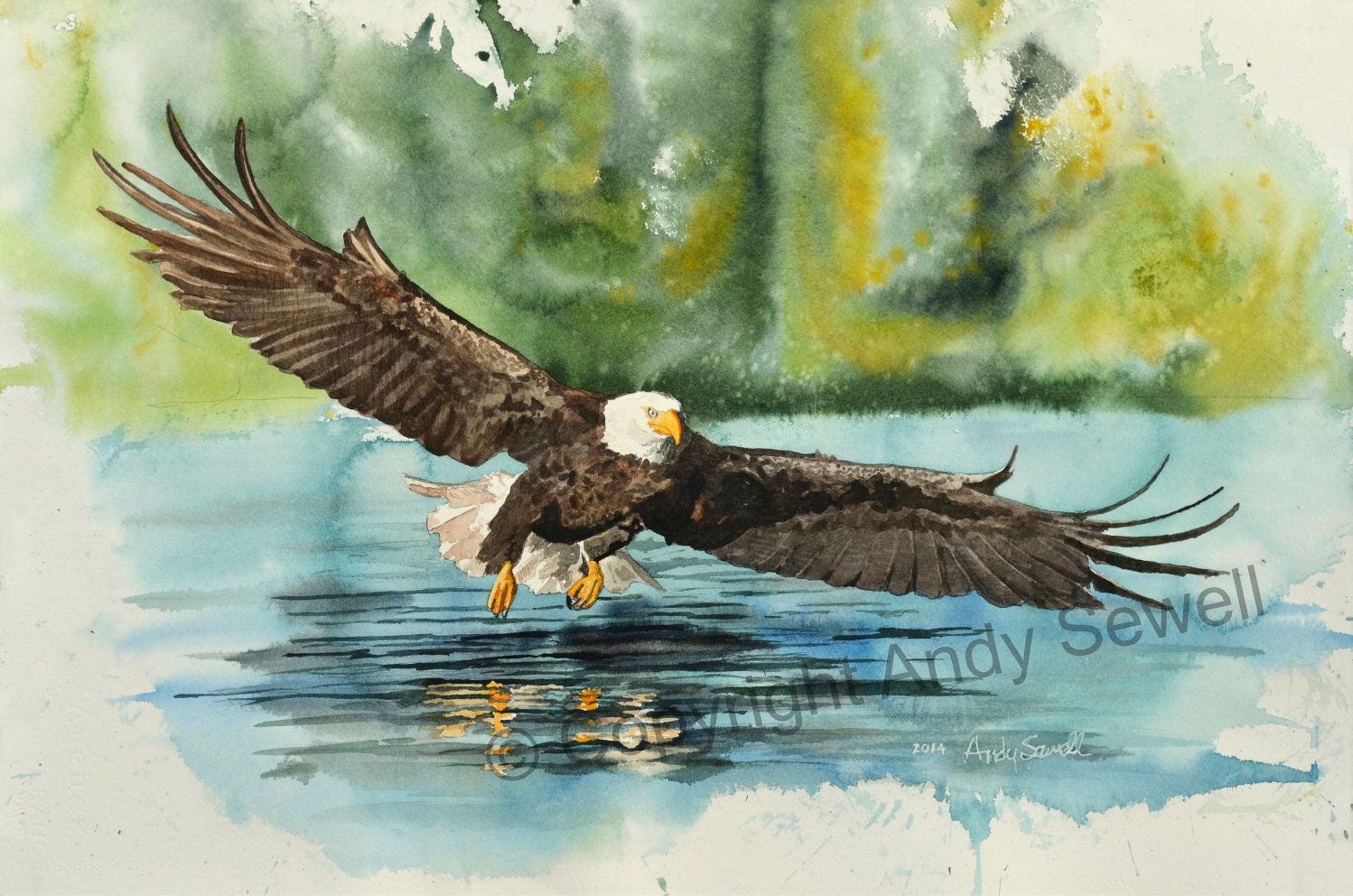This is an impressionist watercolor painting by Andy Sewell, titled and copyrighted in 2014. The composition captures an American bald eagle soaring just above the surface of a serene, sky-blue lake. The eagle, with its striking white head, yellow beak, and white tail feathers, displays its full wingspan majestically. The bird’s reflection shimmers in the darker, central portion of the lake, adding depth to the scene. The eagle’s orange-yellow feet are also faintly reflected in the water. In the background, soft and mottled shades of pastel greens hint at a tree line, blending seamlessly with the blue of the lake to create a tranquil nature scene. The painting’s impressionist style leaves the details slightly fuzzy, allowing the viewer to focus on the ethereal beauty of the moment. The artwork bears a watermark and a signature in white at the bottom, indicating Andy Sewell as the artist.